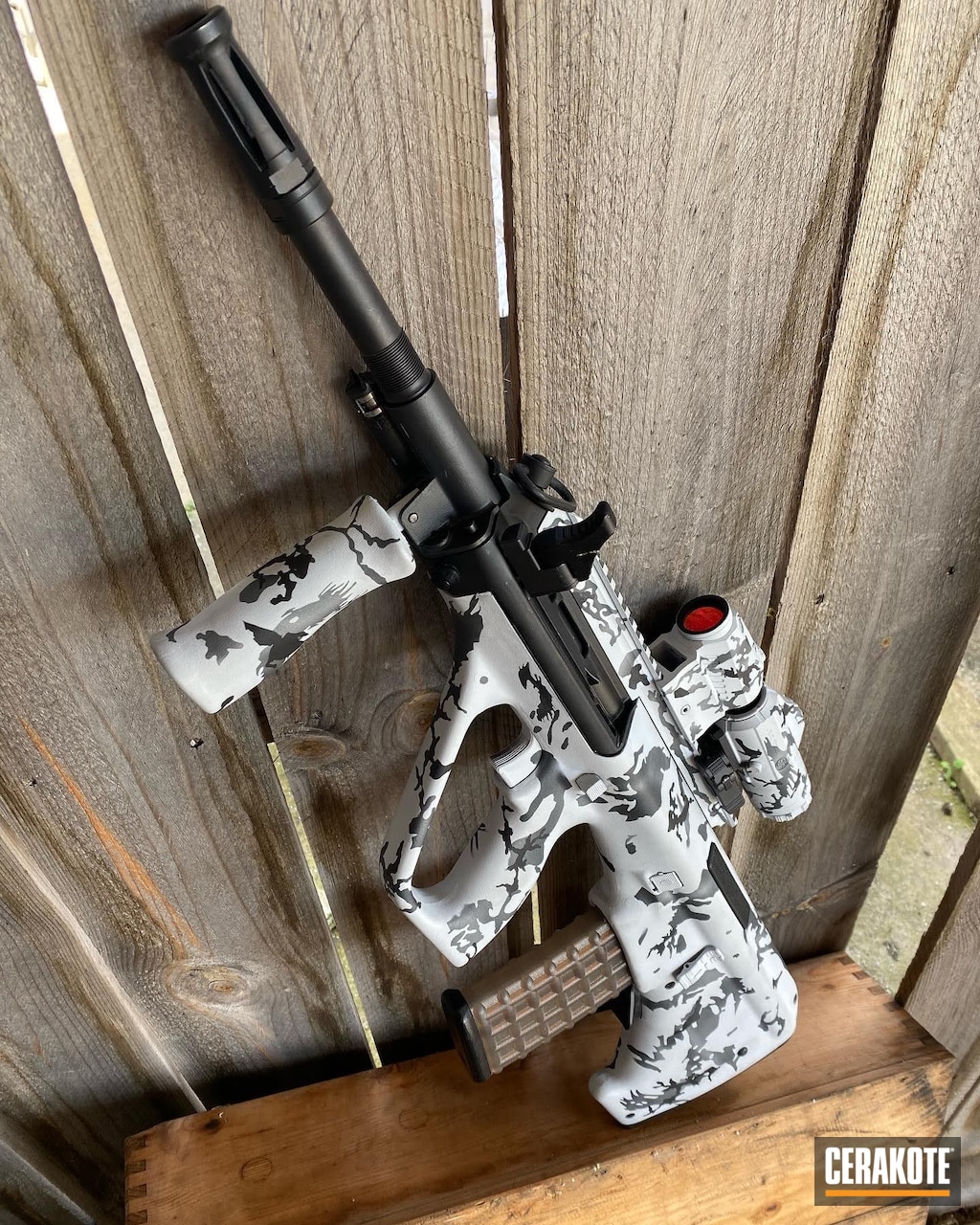This up-close photo features what looks like a combat rifle, potentially an airsoft or paintball gun, distinguished by its white, black, and gray camouflage pattern. The rifle's barrel and tips are a matte gunmetal black, while its stock has a light brown, wafer-like structure, and the trigger is white. The magazine exhibits a light gold hue. The top-mounted scope is camouflaged like the rifle's body and has a red-tinted lens. The rifle, equipped with a harness area for a carrying strap, leans against a wooden picket fence composed of five vertically arranged slabs. It stands on what seems to be an old chestnut box or drawer, with the corners of the drawer visibly jointed. In the bottom right corner of the image, there's a caption that reads "Cerakote," indicating either the brand or additional details about the weapon. There is also a bit of concrete visible in the corner.